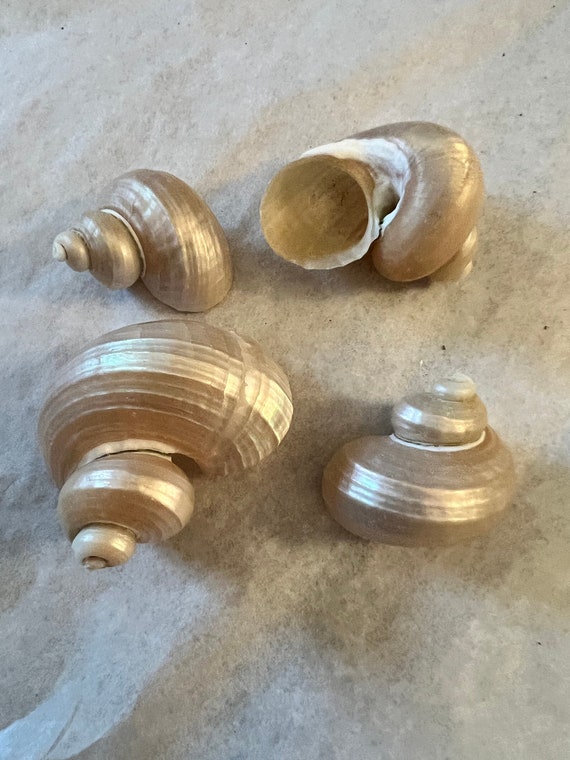The photograph features four unoccupied marine conch shells, each displaying a distinctive spiral shape and notable for their lustrous, iridescent surfaces that resemble pearl or light silver-gray hues. While these shells are of different sizes, with the smallest positioned in the top left corner, all share a polished, glossy appearance that highlights their intricate spiral patterns. The unique button-like ends of each shell add to their decorative charm. Notably, three of the shells are oriented face-down, whereas the one in the top right corner faces upwards, providing a contrasting view. These shells rest atop a stone surface, likely marble or concrete, characterized by a mix of gray tones, adding a sophisticated background to the image.